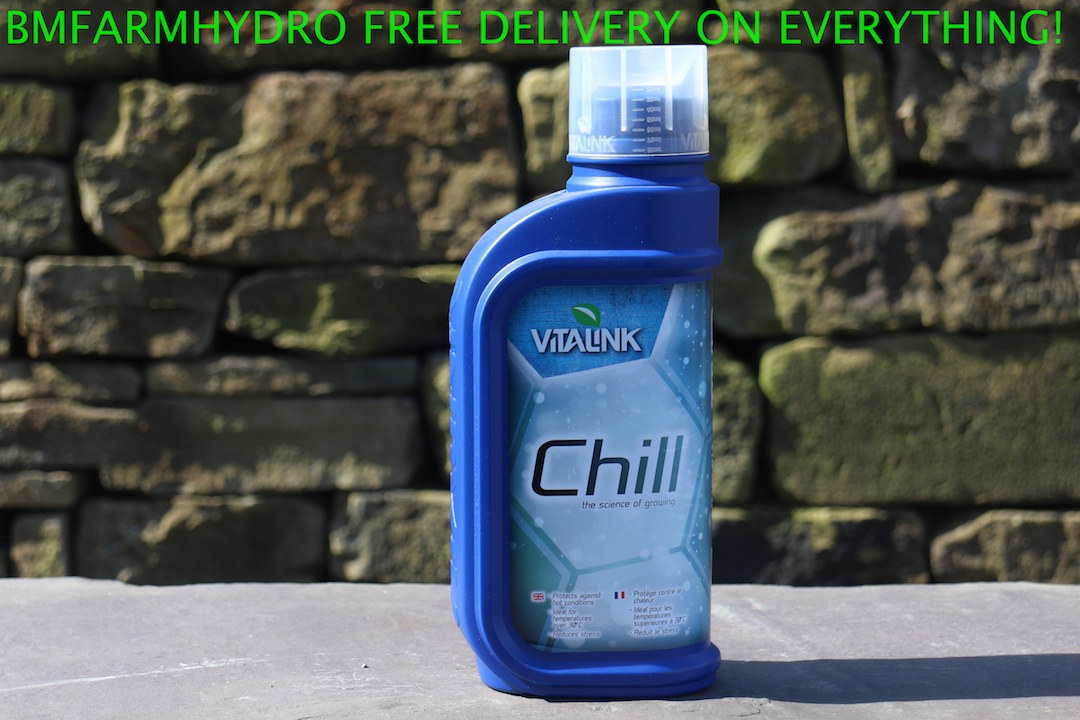The image showcases a wide rectangular advertisement featuring a vibrant blue bottle with a silver cap, prominently displayed on a gray cement-like surface. The background consists of several large, grayish-brown bricks of varying sizes and curviness. The bottle is distinctly curved on the left side and flat on the right, adorned with a lighter blue sticker depicting ice-like hexagons. Central to the label and in italicized blue font is the word "CHILL," accompanied by the phrase "the science of growing." Above this, the brand name "Vitalink" is printed in white, with a green leaf over the "i." At the top of the image, in neon green all capital letters, the text reads, "BM Farm Hydro Free Delivery on Everything!"